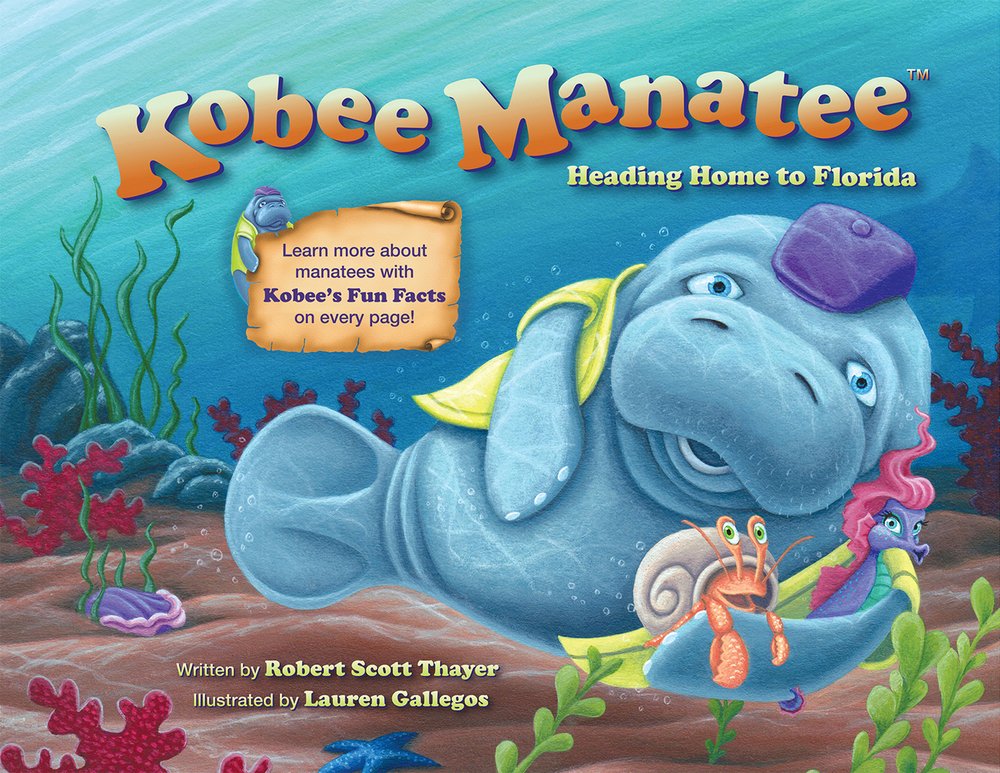This vibrant underwater illustration features a central blue manatee named Kobe, adorned in a cheerful yellow jacket and a playful purple hat. Positioned beneath the orange title "Kobe Manatee" and the yellow subtitle "Heading Home to Florida," Kobe is depicted in a relaxed pose, smiling as he holds a beige scroll that reads, "Learn more about manatees with Kobe's fun facts on every page." This educational message, authored by Robert Scott Thayer and illustrated by Lauren Galagos, emphasizes wildlife awareness.

To the left of Kobe, a grey-shelled red lobster and a charming blue and pink seahorse add lively details, enhancing the underwater scene. The background showcases blue water, green sea plants, starfish, and planktons at the base, creating a rich and immersive oceanic environment indicative of an animated illustration for children.